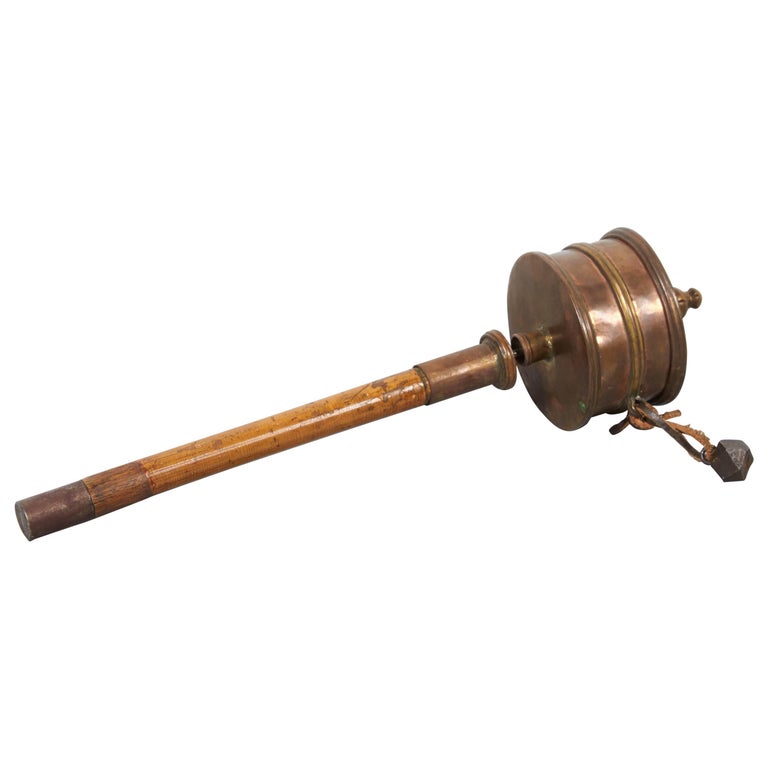In front of me, against a white background, is an antique-looking object that appears to be a rattle or similar instrument. The item features a small, round wooden handle, which is not very big. This handle is capped at both ends by what looks to be copper or brass metal. At the top of the handle, there is a cylindrical metal container, also made of brass or copper. This container has a small lid with an attached knob on top, suggesting it could be opened or adjusted. Additionally, a piece of leather strap is tied to this cylindrical container, holding a small round metal piece. This combination of wood and copper metal gives the entire object an old-fashioned, possibly handcrafted appearance, reminiscent of something one might find on Antiques Roadshow. The leather strap and metal piece suggest it could produce a rattling sound, hinting at its potential use as a historical rattle or toy.